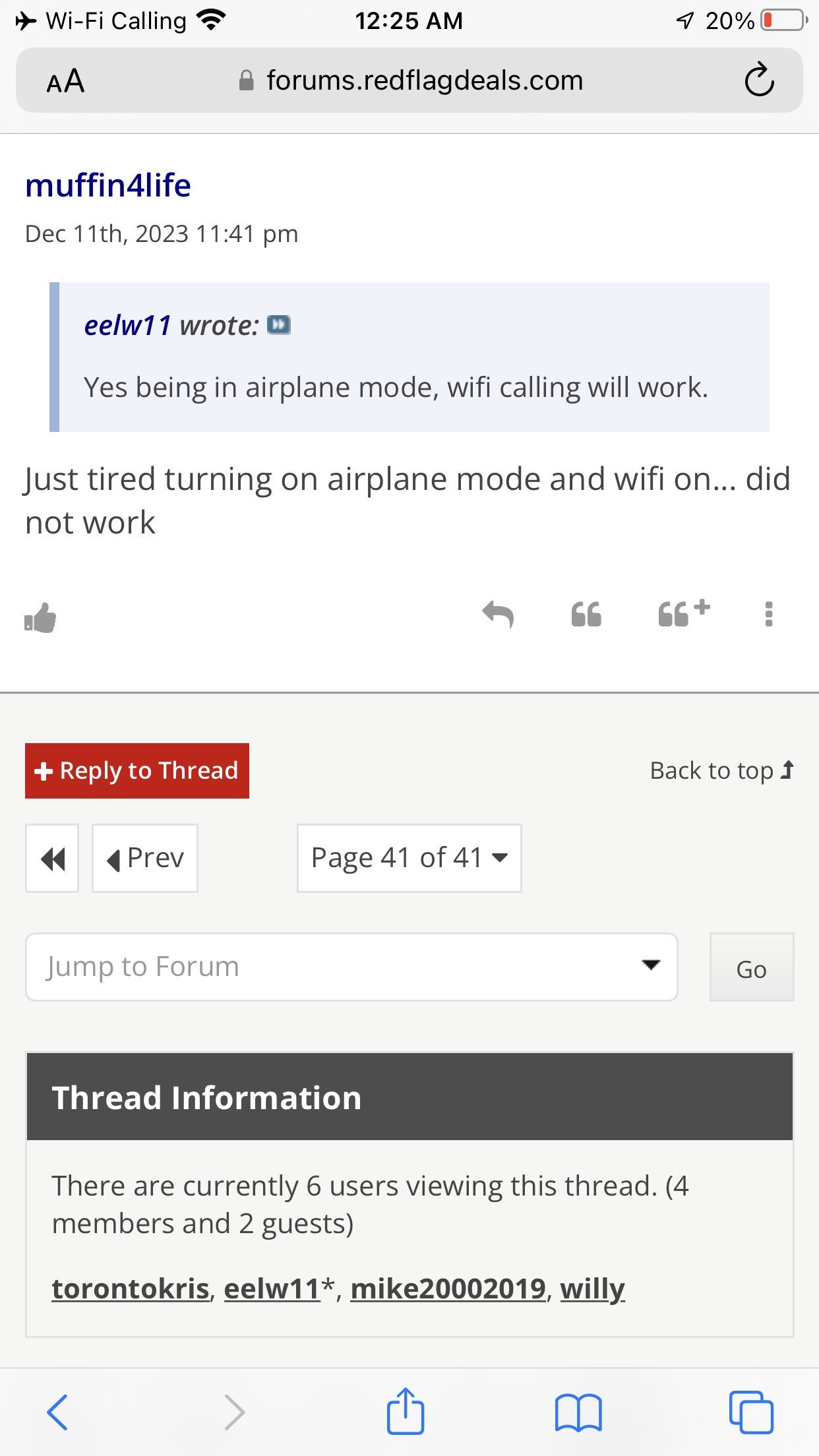A mobile screenshot captured at 12:25 AM displays several details. The top of the screen shows 'Wi-Fi calling' on the left and a battery percentage of 20% on the right. The search bar indicates the website 'forums.redflagdeals.com'. Below, a post is highlighted from a user named 'Muffin for Life' with the timestamp December 11, 2023, at 11:41 PM. The post quotes another user, 'eelw11', who mentioned that Wi-Fi calling should work in airplane mode. 'Muffin for Life' responds stating, "Just tried turning on airplane mode and Wi-Fi on... did not work." Adjacent icons include options for a thumbs-up, reply, quote, bookmarks, and additional settings. The bottom section features navigation controls like 'Reply to Thread', page navigation arrows, a current page indicator (41 of 41), and a dropdown menu labeled 'Jump to Forum' with a 'Go' button. Further below, a grey box marked 'Thread Information' in white text notes that there are currently six users viewing the thread: four members (Toronto Chris, ELW11, Mike2019, and Willie) and two guests.